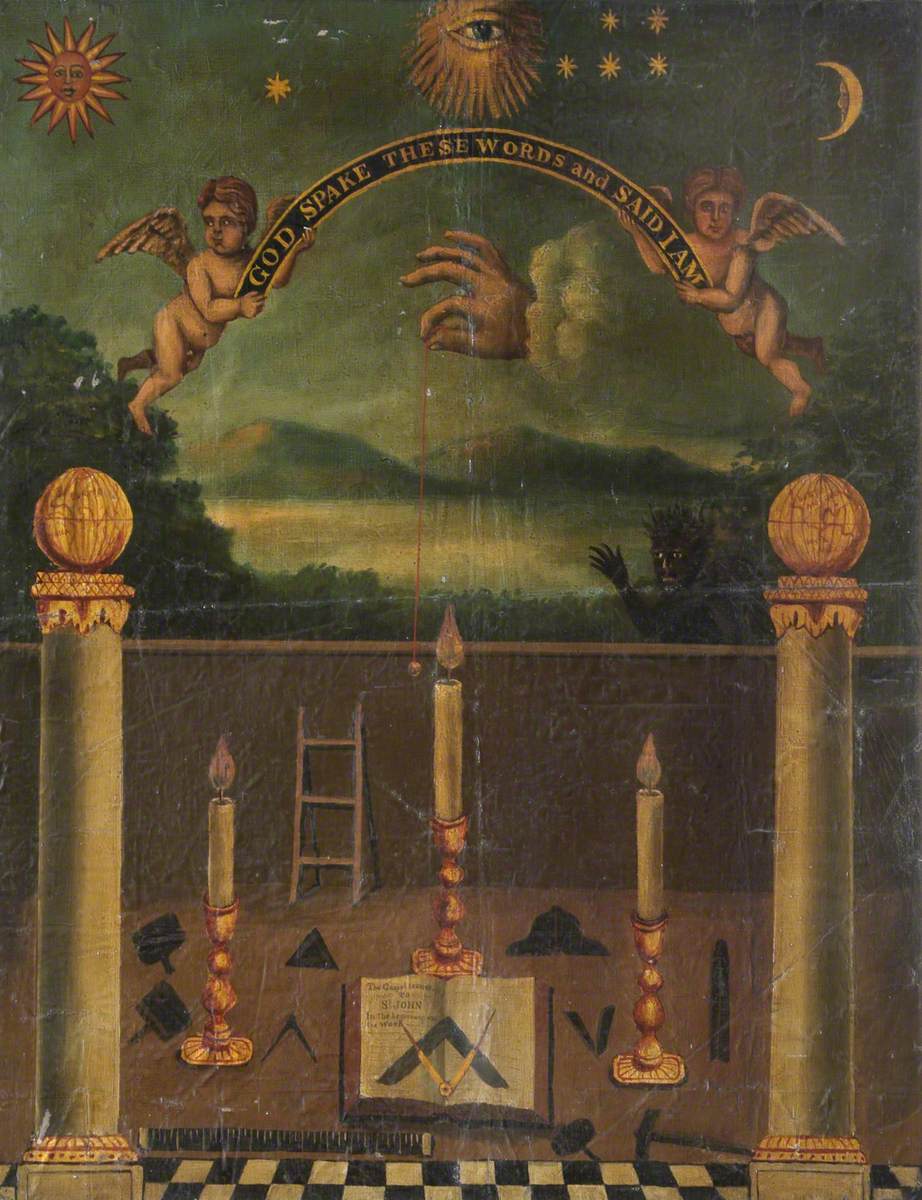This detailed painting, evidently aged and damaged with scratches, bends, and folds, depicts a rich tapestry of symbology. At the top left corner, an anthropomorphized sun gazes out, juxtaposed by a similarly humanized crescent moon on the top right. Between these celestial bodies is an eye emanating rays of light, surrounded by a scattering of stars. Below, two cherubic angels, hovering in mid-air, hold a curved banner reading "God spake these words and said, I am." Emerging from clouds beneath them is a disembodied hand, poised as if holding a thread with a ball. 

The lower half of the painting features two columns, each crowned with a globe-like sphere, flanking an open book resting amongst three lit candles. In the backdrop sits a minimalistic ladder with three steps, suggesting a climb or ascension. The painting's base is adorned with a checkerboard floor pattern. Adding an eerie note, a silhouette of a figure, perhaps a demon, subtly blends into the middle right side of the scene. Notably, the artist left no visible signature or initials on this intriguing, mystical artwork.